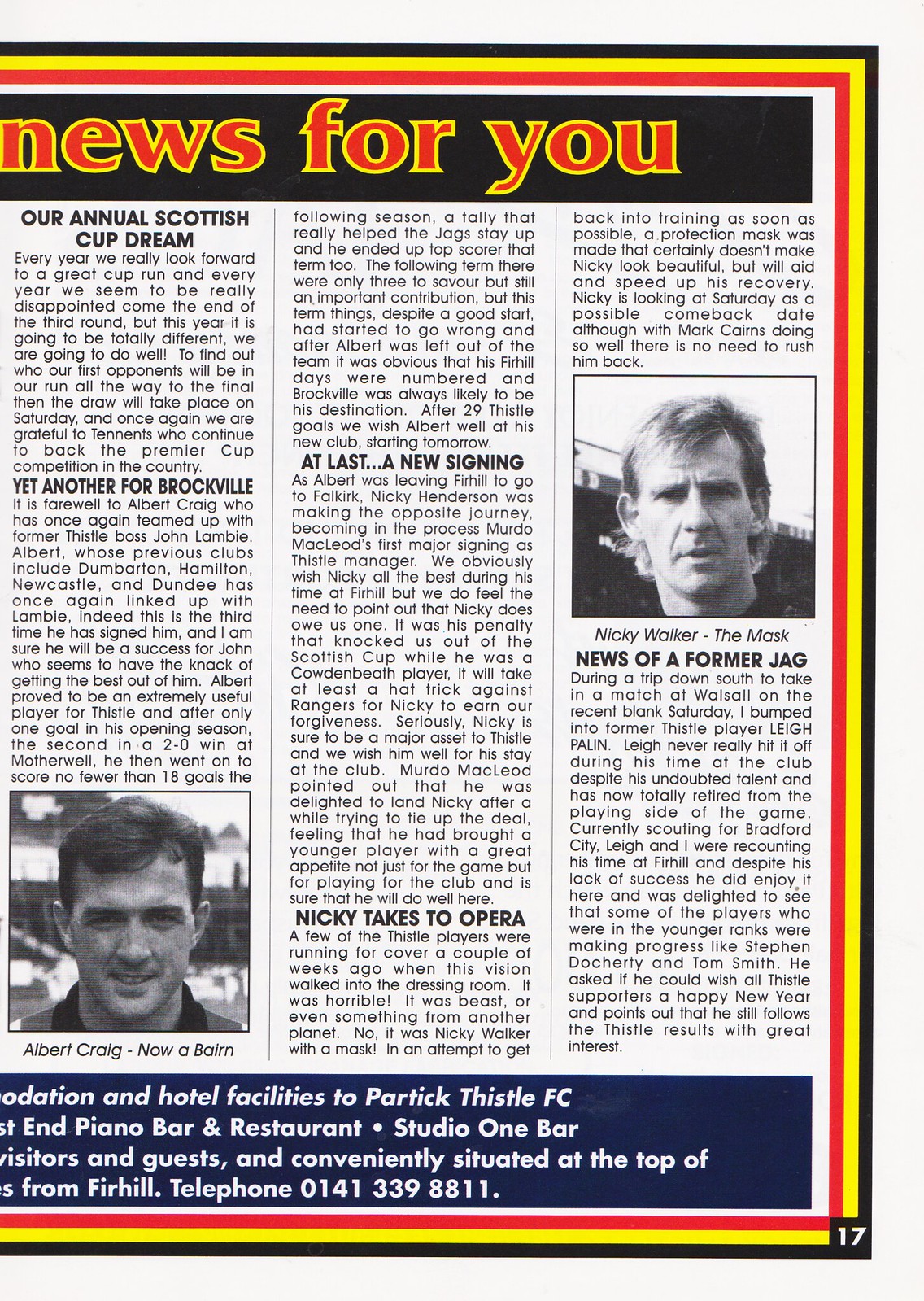The image is a vertical, rectangular magazine page with a predominantly white background. It features a three-bordered design with the innermost border in red, followed by yellow, and the outermost border in black, with the left side cut off. At the top and bottom of the page, black horizontal bars stretch across; the top bar displays "News for You" in red text with a yellow outline, while the bottom bar in white text advertises hotel facilities linked to Partick Thistle FC, including a Piano Bar and Restaurant, Studio One Bar, and a contact number: 0141 339 8811.

The magazine page is divided into three vertical sections filled with black text, largely discussing the Scottish Cup Dream. The top of the first section reads "Our Annual Scottish Cup Dream," followed by paragraphs and the headline "Yet Another for Brockville." At the bottom of this section, there's a photograph of a man labeled Albert Craig, described as "now a Bairn."

The second section continues the discussion from the first and introduces a new topic with the headline "At Last, A New Signing," followed by another paragraph and the headline "Nikki Takes to Opera," which continues into the third section.

The third section contains a central photograph of another man, labeled Nikki Walker, "the mask," with a subheading "News of a Former Jag." The bottom right corner of the page is marked with the number 17. Additional smaller text beneath the photographs and headlines offers further details on the topics discussed.